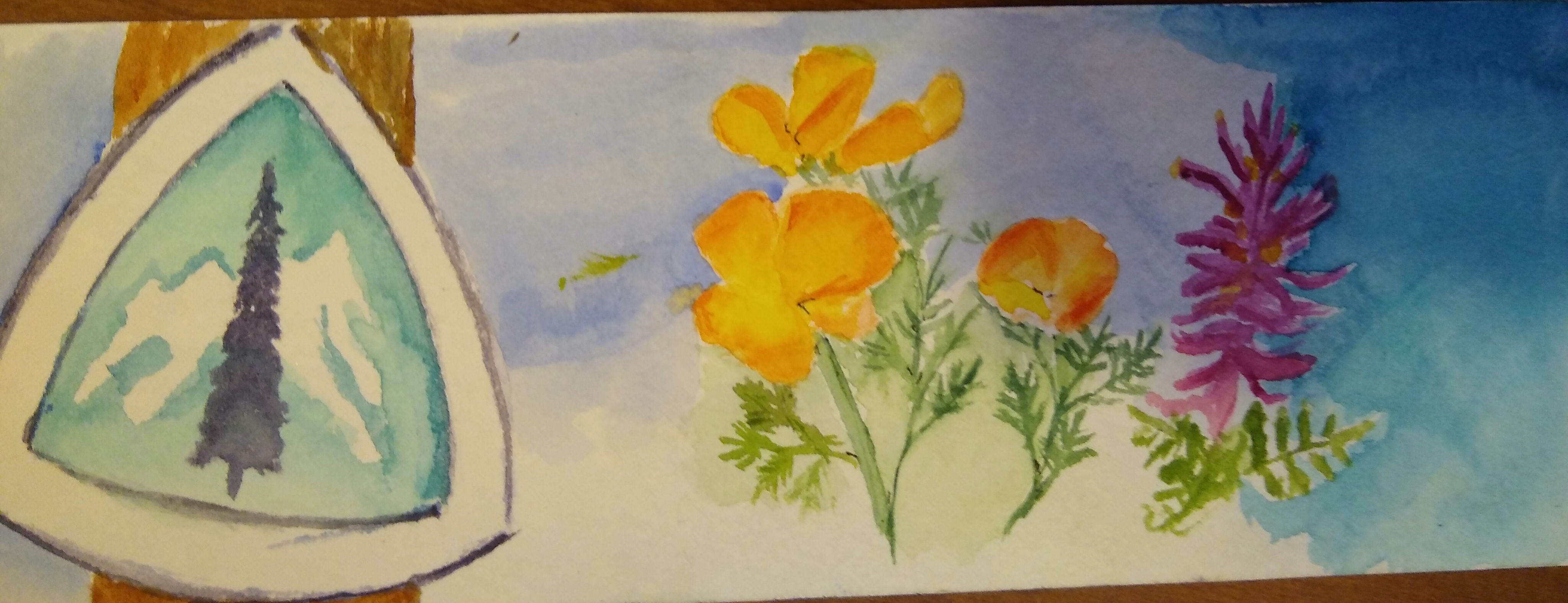This captivating artwork is a multi-medium creation portraying an array of intricate flowers against a dynamic background. The background transitions seamlessly from blue to blue-green to purple, creating a dreamy, watercolor-like effect. On the left side, there's an intriguing element that possibly utilizes crayon, depicting a pole and a tree symbolizing a forest, with a brown hue that stands out prominently. The flowers themselves showcase a combination of artistic techniques; the intricate details of the stems, buds, and petals suggest the use of oil paint, while the flowering parts might have been rendered with watercolor. On the right, a stunning purple flower captures attention, exhibiting what appears to be a blend of watercolor and other paint mediums. The bottom of the background subtly shifts to an off-white shade, grounding the vibrant and diverse elements of the piece.